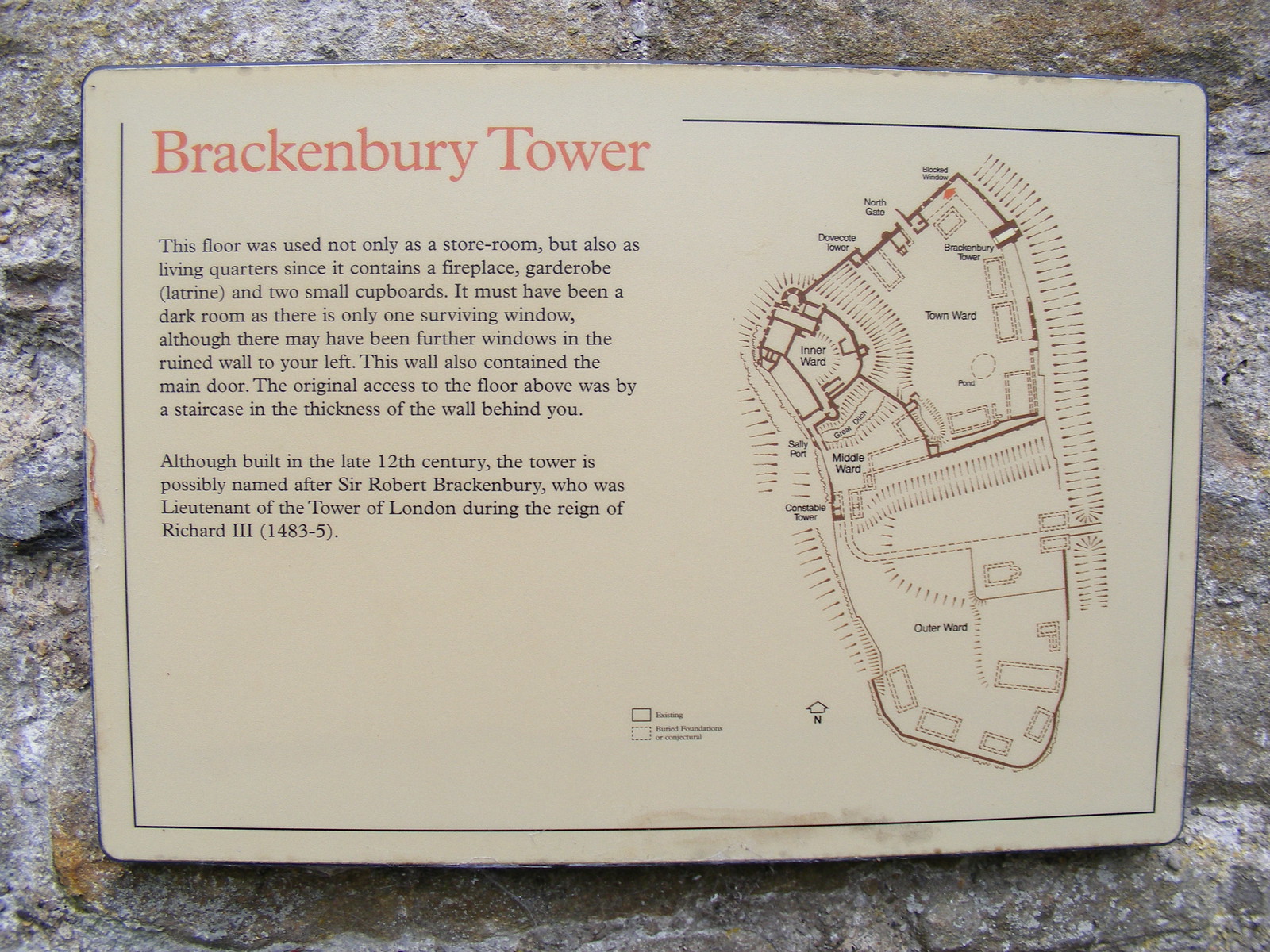The photograph, taken outdoors during the daytime, captures a rectangular metal placard on a stone wall with varying shades of gray, white, blue, and orange tones. The sign itself is tan-colored and slightly worn at the edges, particularly in the upper left corner. The top left of the sign features large red text reading "Brackenbury Tower". Below, black text explains that the floor was used both as a storeroom and living quarters, containing a fireplace, guardrobe, latrine, and two small cupboards. The text notes that the room must have been dark due to a single surviving window, though additional windows may have existed in the now-ruined adjacent wall, which also held the main door. Access to the floor above was originally via a staircase built into the wall's thickness behind the viewer. The sign mentions that although the tower was built in the late 12th century, it might be named after Sir Robert Brackenbury, lieutenant of the Tower of London under Richard III from 1483 to 1485. On the right side of the placard is a hand-drawn, kidney-shaped map of Brackenbury Tower, labeled with various sections of the tower and nearby features, including a blocked window, wards, gates, ponds, and ditches. An arrow at the bottom of the map indicates north.